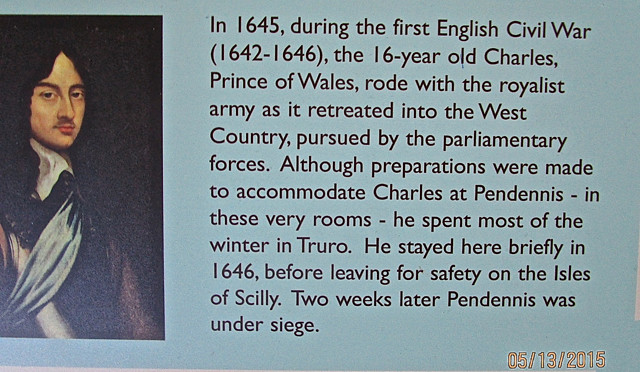The image shows an informational sign with a light blue background and a date in the lower right corner reading "05-13-2015." On the left side is a painting of a man dressed in old-fashioned clothing, consisting of a dark burgundy tunic with a blue sash running from his shoulder to his waist. The man has long black hair. To the right of the painting, there is a column of black text that reads: "In 1645, during the First English Civil War, 1642-1646, the 16-year-old Charles, Prince of Wales, rode with the Royalist Army as it retreated into the West Country, pursued by the Parliamentary forces. Although preparations were made to accommodate Charles at Pendennis, in these very rooms, he spent most of the winter in Truro. He stayed there briefly in 1646 before leaving for safety on the Isles of Sicily. Two weeks later, Pendennis was under siege." The image appears to be describing an event from the First English Civil War, focusing on the role of Charles, Prince of Wales, during that time.